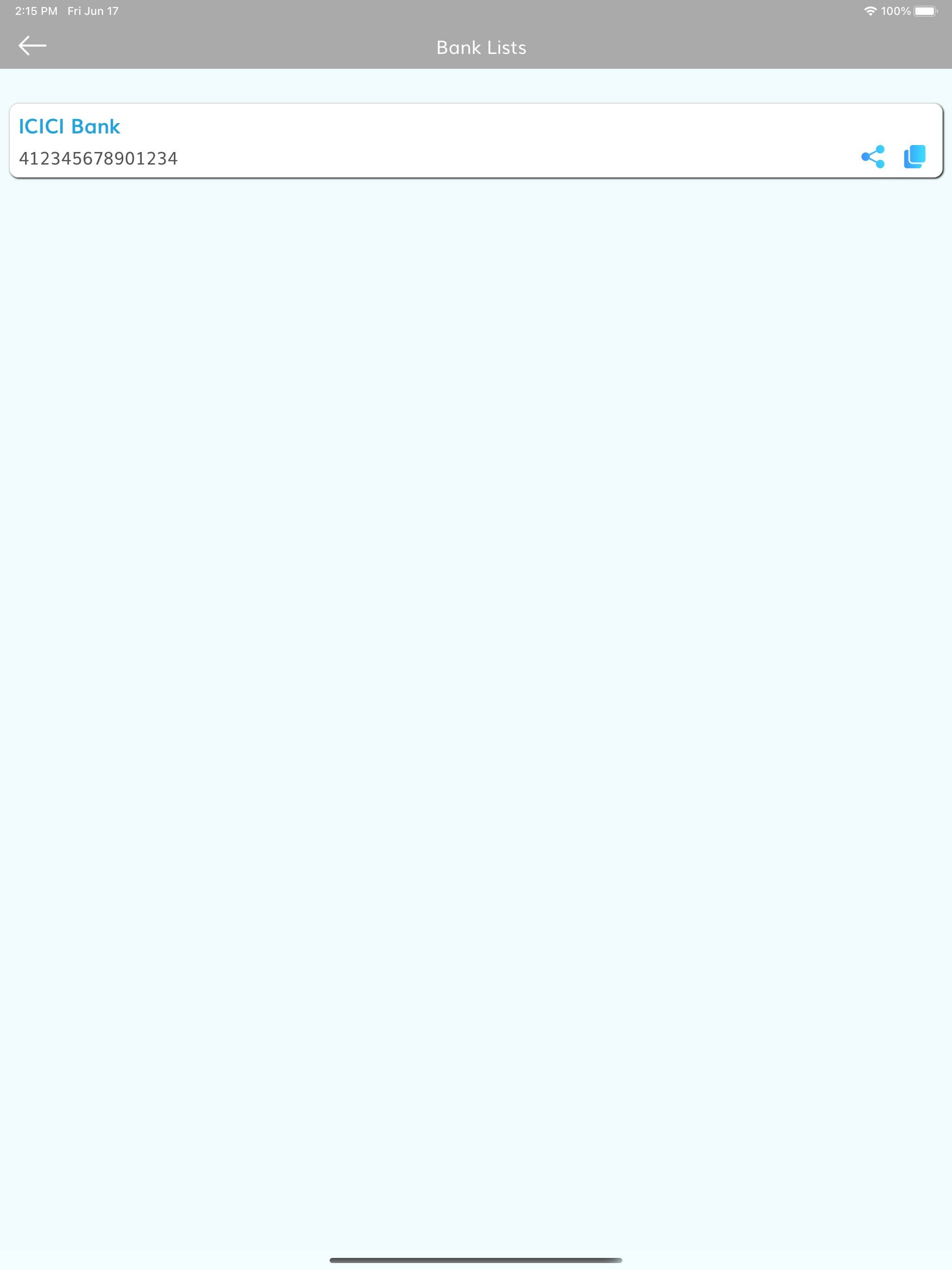A detailed caption for the given image could be:

"This screenshot, taken from a tablet in landscape mode, displays a banking application interface. The header of the screen is dark grey, featuring the title 'Bank Lists' centered in white text, with a left-pointing arrow located at the far left. The top left corner of the header shows the current time and date, while the top right corner displays icons for Wi-Fi connectivity, battery percentage, and the battery icon. Below the header, the page body has a light blue background. Dominating the top portion of the page is a long white rectangle that spans the width of the screen, containing the name 'ICICI Bank' in bold blue font. Directly beneath this is an account number. To the right of the account information are two icons, both in blue: one for sharing and one for copying the account details. At the very bottom of the screenshot, a thin grey horizontal line is centered across the width of the screen. The rest of the page below the white box is blank and appears unused."